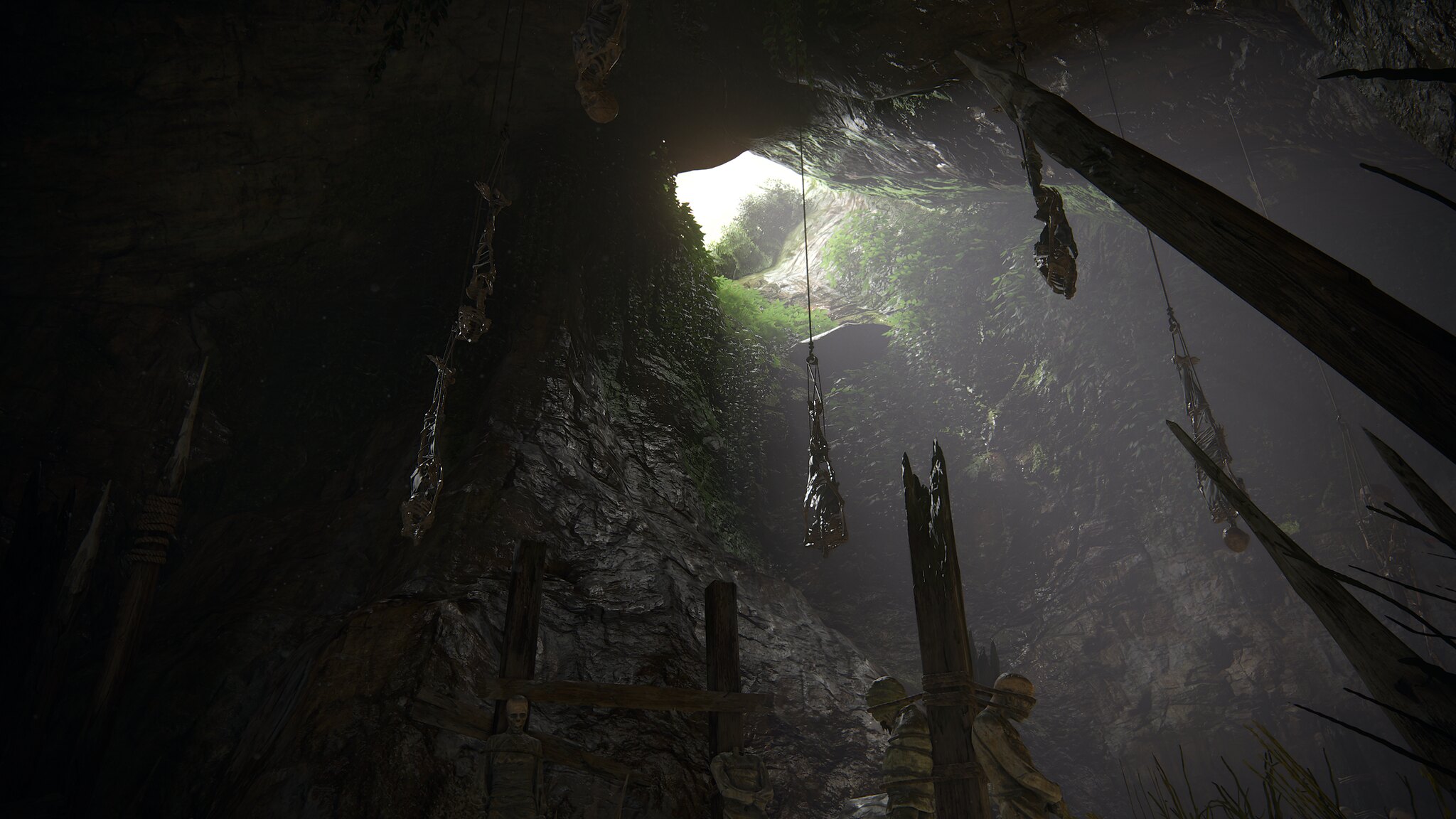Inside the dimly lit cavern, a large natural skylight at the top allows sunlight to stream in, revealing a tree perched at the edge of the opening. The cavern walls, composed of rugged stone, are adorned with patches of greenery. Suspended from the ceiling, two individuals, now just skeletons, hang upside down by ropes, swaying slightly. Below them, the cavern floor is lined with sharp stone spikes or pillars. At the bottom, several figures, possibly tied-up individuals, are visible, suggesting that this pit served as a grim site where people were hurled down and left to perish upon the lethal spikes.